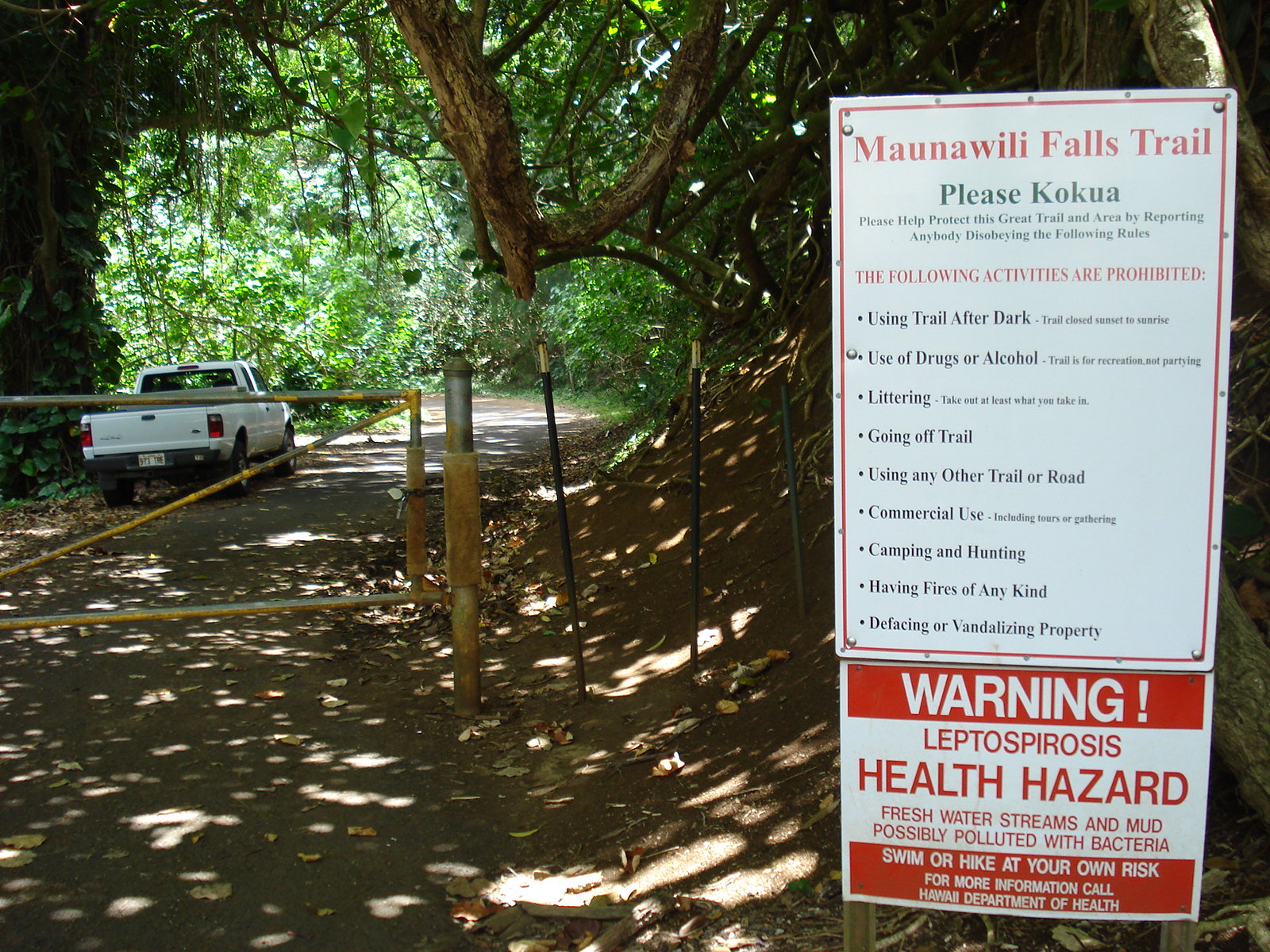This photograph captures the entrance to the Mauna Wili Falls Trail. Dominating the scene is a closed yellow gate with a white pickup truck parked just beyond it. To the left of the frame, the trail begins, winding its way into a dense area filled with brush and trees. Adjacent to the trail is a prominent sign, white with red and black text. In red, the sign announces the name of the trail: "Mauna Wili Falls Trail." Below, in black text, visitors are urged to "please help protect this great trail and area by reporting anybody disobeying the following rules." It lists several prohibited activities in black text: using the trail after dark, using drugs or alcohol, littering, going off trail, using any other trail or road, commercial use, camping and hunting, having fires of any kind, and defacing or vandalizing property. Beneath this, another conspicuous red and white sign issues a stark warning: "Health hazard, freshwater streams and mud possibly polluted with bacteria. Swim or hike at your own risk." The right side of the image also reveals a lush backdrop of trees, adding to the natural and somewhat foreboding atmosphere of the area.